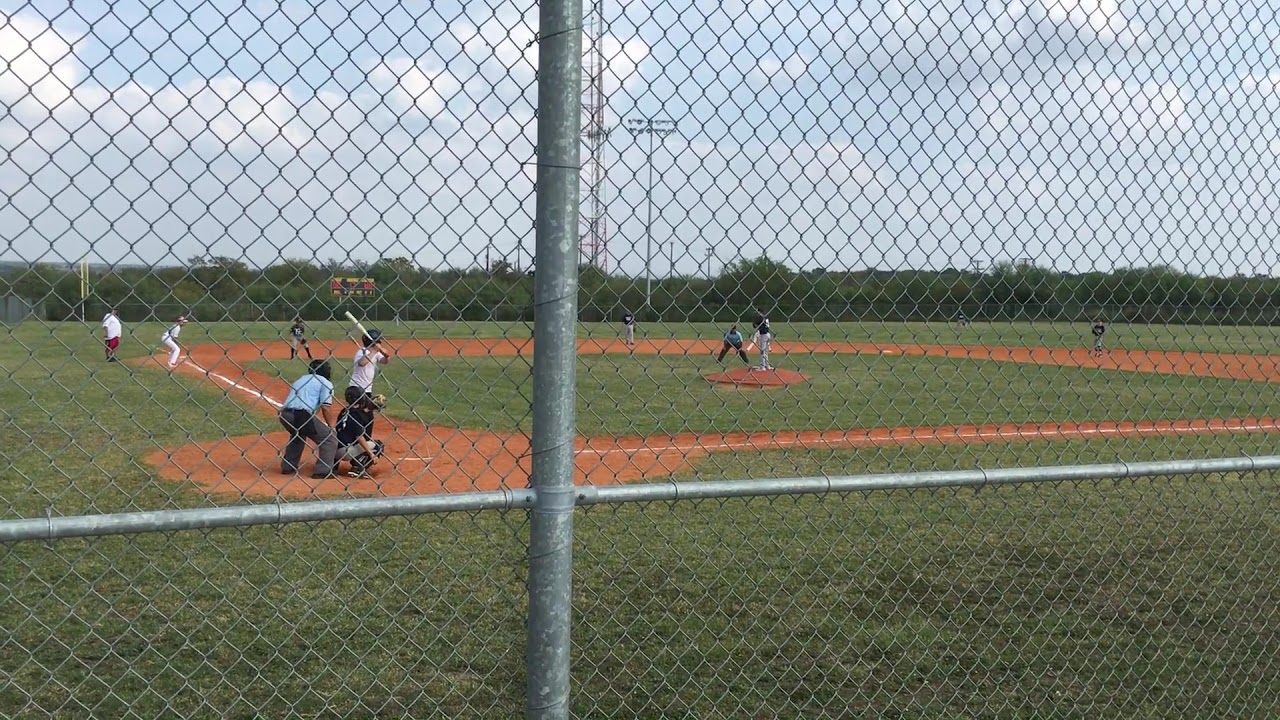This photograph captures an active baseball game in progress on a large baseball field, viewed from behind a metallic silver chain-link fence. Prominently featured are the green grass covering the outfield and the brown dirt outlining the infield, marked with lines delineating home base, first, second, and third bases, and the pitcher's mound at the center. In the foreground, the umpire, dressed in a light blue shirt and gray pants with protective gear, stands behind the squatted catcher, both closely observing the batter. The batter, wearing a white jersey and helmet, grips a bat, ready to face the incoming pitch. Other players are visible, positioned strategically across the field, while a runner waits on third base, anticipating his chance to dash home. The background beyond the field features a row of trees, stadium lights, a large tower, and a blue sky adorned with white clouds. The scene appears serene with no visible audience, suggesting it might be taking place in a park.